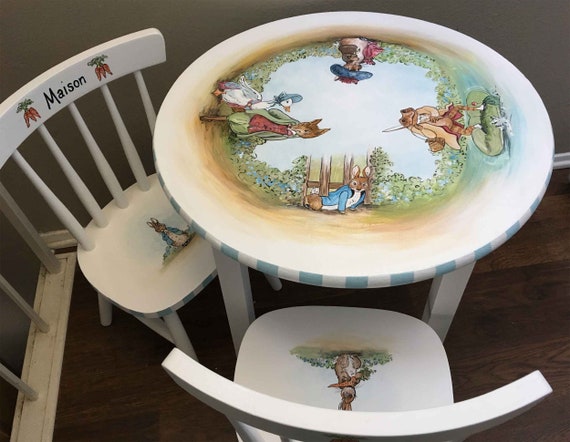A charming children's dining set is meticulously illustrated with scenes from Peter Rabbit. The round, white table features an alternating white and blue rectangle trim around the edge and showcases four Peter Rabbit characters, one at each cardinal point. Positioned northward is a rabbit wearing a blue jacket. To the east, a character stands on a fish, holding a fishing rod. On the west side, a fox or wolf in a green suit and red shirt converses with a goose wearing a blue bonnet. The south of the table reveals another rabbit, this one sporting a large-brimmed blue hat.

Interspersed among these characters are lush green plants and various outdoor elements such as gates and fences, creating a whimsical garden setting. Two wooden chairs, each with the same blue and white trim, accompany the table and feature additional Peter Rabbit illustrations. The chair on the left bears the name “Mason” flanked by bunches of three carrots, indicative of its personal touch. Each chair is adorned with its own unique character illustration. The set is set against an older wooden floor and surrounding poles, contrasting with the fresh and intricate paintings on the furniture, making the dining set stand out vividly.